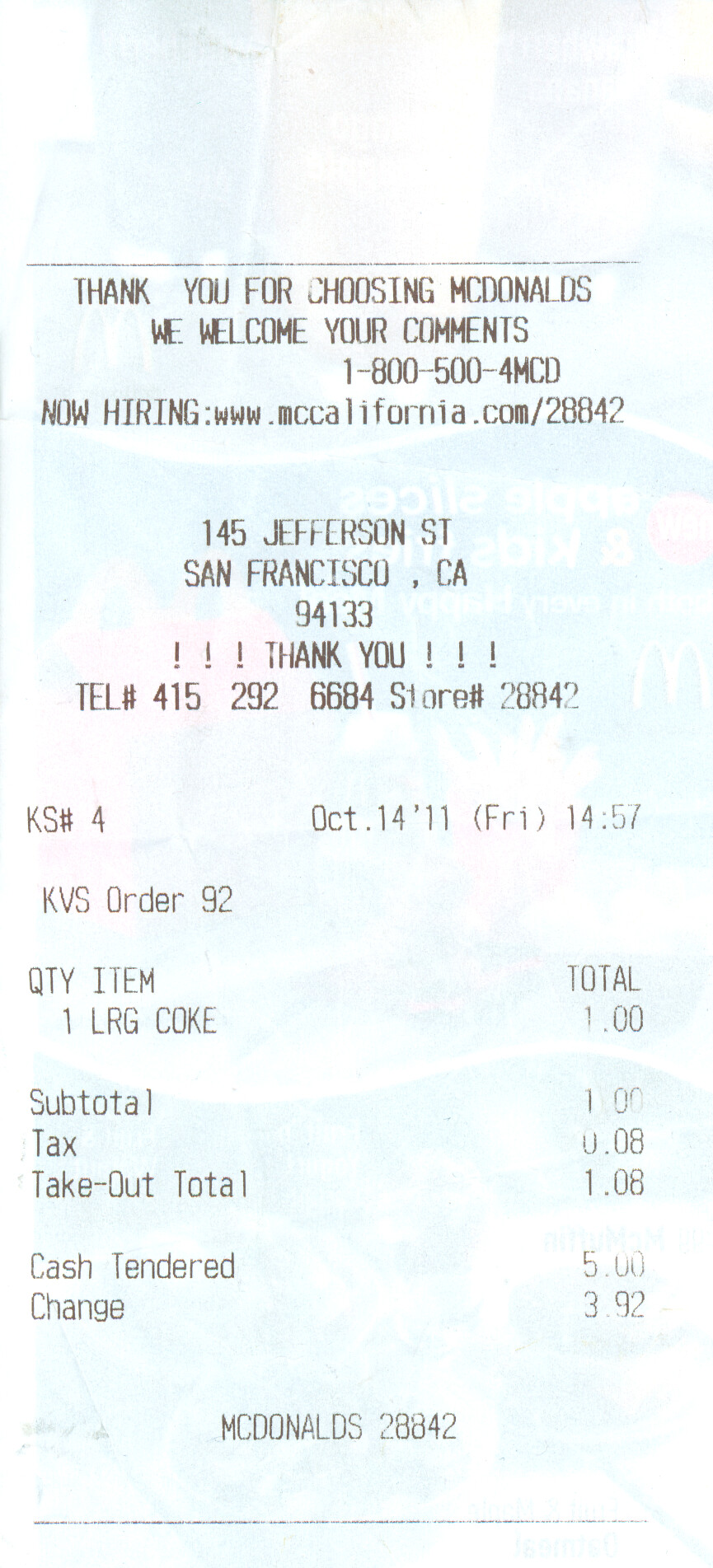A detailed caption for the image:

"This is an image of a McDonald's receipt from the location at 145 Jefferson Street, San Francisco, CA 94133. The header of the receipt includes the message 'Thank you for choosing McDonald's. We welcome your comments.' and provides the customer service number '1-800-504-MCD' alongside a notice for job opportunities at 'www.mccalifornia.com/28842.' The store number is identified as '28842,' and the receipt indicates it was printed on October 14. 

The specific order details show that 'KVS order 92' was placed on a Friday ('Fry') at 14:57 (2:57 PM) and contained one large Coke (LRG Coke) priced at $1. The subtotal comes to $1 with an additional tax of $0.08, bringing the total to $1.08. The payment section indicates 'cash tendered' as $0.00 and 'change' as $3.92, perhaps indicating an error.

The footer of the receipt reiterates the store number '28842' and is bordered by straight lines at the top and bottom. The document itself is white with black text, providing clear visibility of the transactional details."